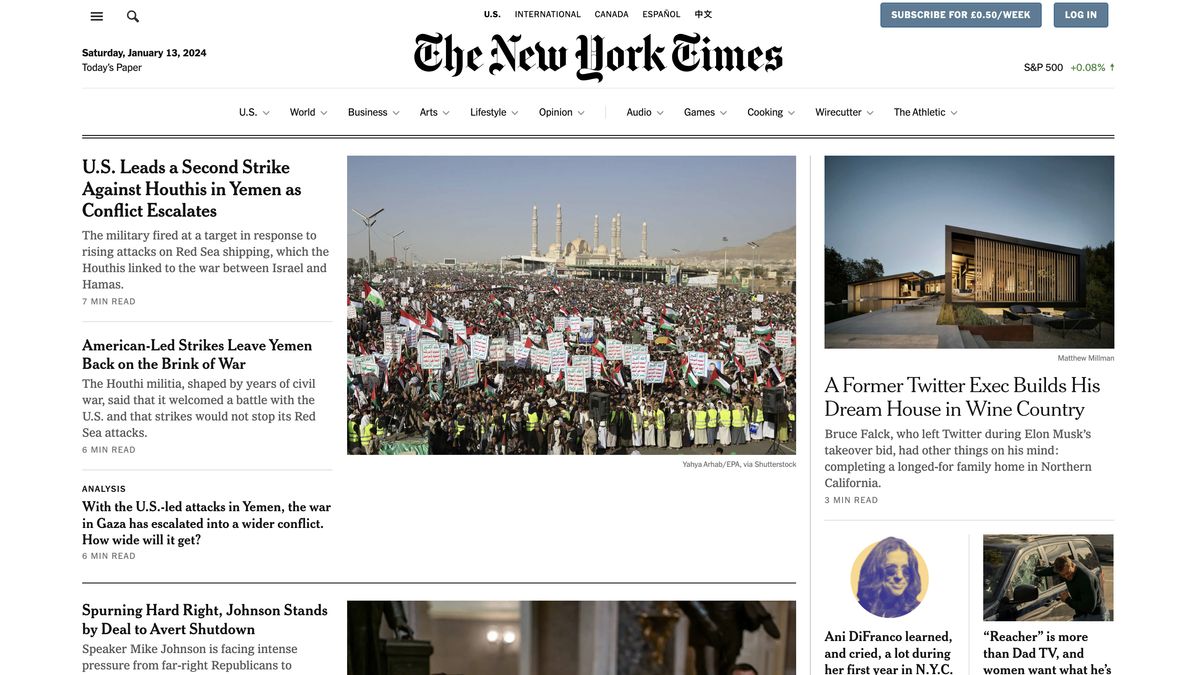This is a screenshot from The New York Times website, captured on Saturday, January 13, 2024. The headline story highlights a significant event in Yemen, showing tens of thousands of people gathered in front of a religious building during the day, holding placards and signs. The white minarets of the building are visible in the background. The headline reads: "U.S. Leads a Second Strike Against Houthis in Yemen as Conflict Escalates." The subtext explains that the military operation targeted Houthis in response to rising attacks on Red Sea shipping, which have been linked to the ongoing conflict between Israel and Hamas.

Additionally, there are other news stories featured on the page. One noteworthy article is about a former Twitter executive who has built his dream house in wine country. The accompanying photograph showcases a modern, luxurious home set amidst a lush green landscape under a clear blue sky.